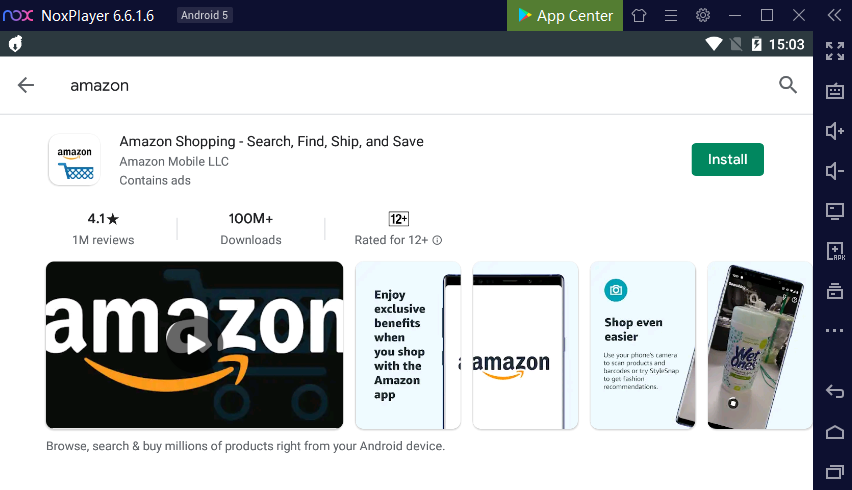A screenshot taken from a mobile device or tablet captures the Google App Store interface. The Google Play logo is visible in the upper-middle right of the screen, confirming the platform. The main focus is on downloading Nox Player, version 6.6.1.6 for Android 5, with the text and Nox logo (N-O-X) displayed prominently in the upper left corner. A grey bar beneath the logo hints that the screenshot may be from a cell phone, reinforced by the timestamp (15:03), battery percentage, and Wi-Fi signal strength in the upper right corner of the image.

Further down the screen, the user appears to be attempting to download the Amazon Mobile LLC app, recognizable by the standard Amazon logo featuring a blue shopping cart. Adjacent to the app details is an install button, green with white text. Information about the app's rating, download count, and a link to a video overview can also be seen, providing additional context on the app's functionality.